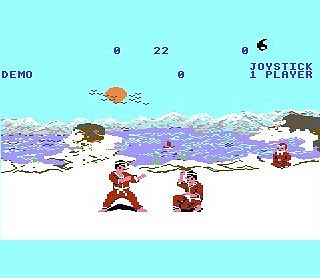This image captures a screenshot from an 8-bit 2D fighting video game, reminiscent of classic arcade-style side-scrollers. The scene is set against a blue background that may represent either sky or water, adding a vivid contrast to the visual. In the foreground, two characters stand poised for battle on what appears to be a snow-covered ground. Each character is clad in traditional martial arts outfits; one wears a turquoise kung fu uniform while the other dons a burgundy one. 

Behind the fighters, a figure is seated, possibly indicating an impending fight. The scene includes a digital interface with the text "demo" and "joystick one player" displayed prominently, suggesting that this is a demonstration mode screen. Additionally, there is a depiction of the sun with birds flying across it, adding a touch of detail to the background. Various numbers are also visible, though their specific purpose is unclear in this isolated screenshot. Overall, the image exudes the nostalgic charm of vintage video games.